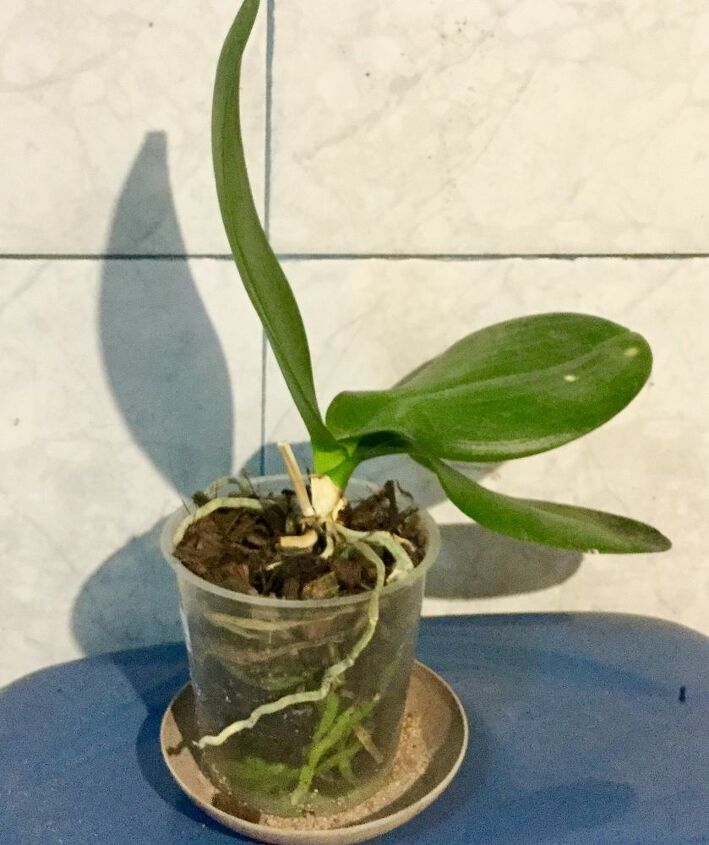The image is a detailed color photograph depicting a plant growing out of a clear plastic cup. The cup is filled with soil and wood chips, revealing a network of white and green roots inside. The plant is rooted in a whitish base, from which three long, oblong green leaves extend—one upright and two arching to the right. The cup is positioned in a small, beige saucer, which rests on a blue-gray surface. In the background are large ceramic white tiles with dark gray veining, forming a cross pattern where their corners intersect. The scene is brightly lit, casting a prominent shadow of the plant to the left, suggesting strong sunlight from the upper right.